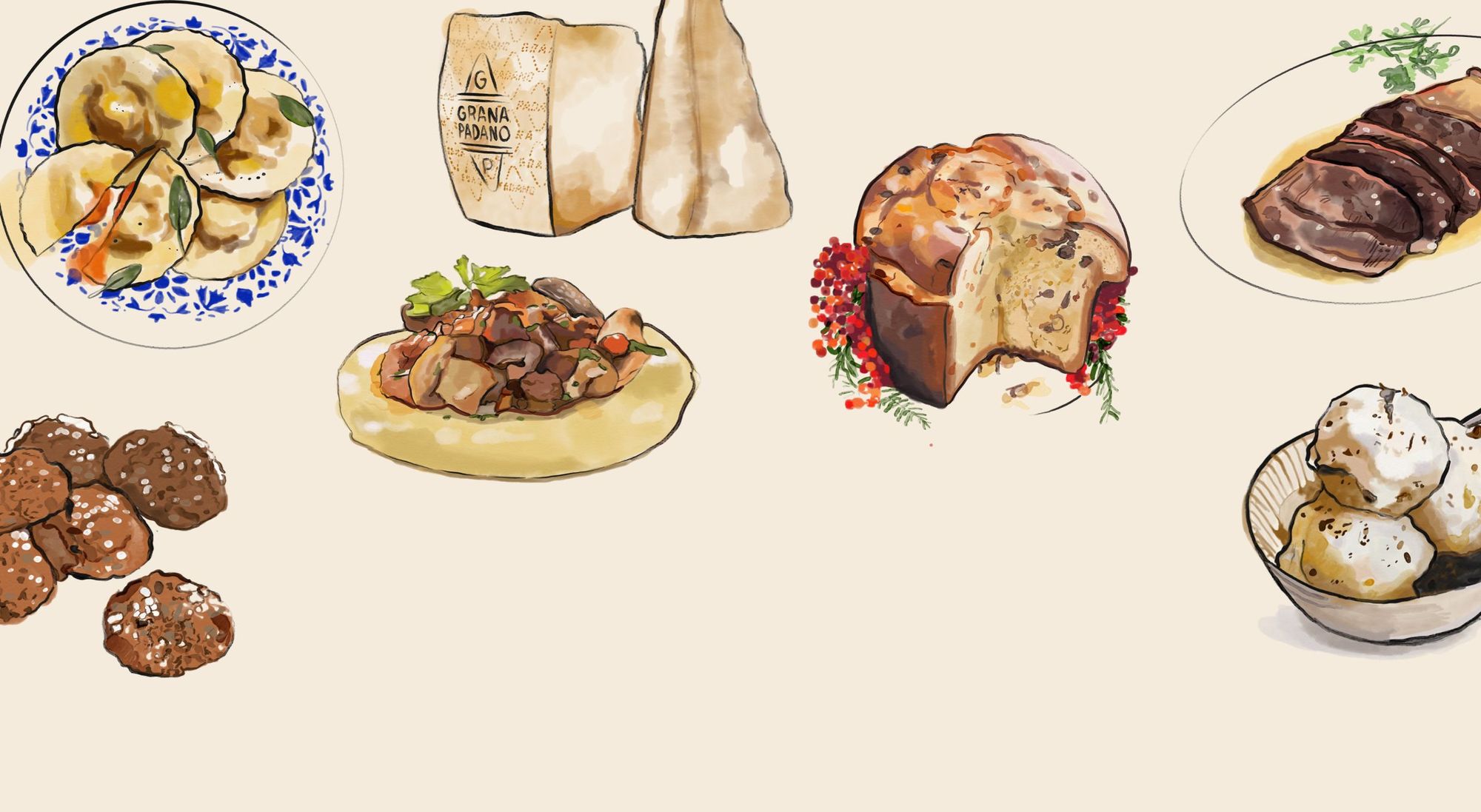This hand-drawn illustration depicts an assortment of various foods, all laid out on a tan background that resembles a tabletop. Central to the image is a cake adorned with red flowers and greenery, with a triangular slice missing. Above the cake, a platter of sliced meat is garnished with some greenery. To the left, a tan bowl contains speckled items resembling potatoes. Close by, in the top left corner, sits a plate of pierogies. Below these pierogies are round items that could be meatballs or cookies. Nearby, two bags labeled "grena, pandano" lie adjacent to a pretty dish decorated with blue flowers, holding what appears to be large mushroom heads or a similar dish. Adding to the variety, there’s a bowl that seems to contain a stew-like substance, as well as a flat bowl with what might be a dollop of hummus topped with meat. The top right corner features another dish of sliced meat, and just below it, a bowl containing what looks like scoops of ice cream or snowball cookies. Scattered across the scene are other baked goods, possibly apple fritters, cookies, and cupcakes, all contributing to the realistic and colorful depiction of food.